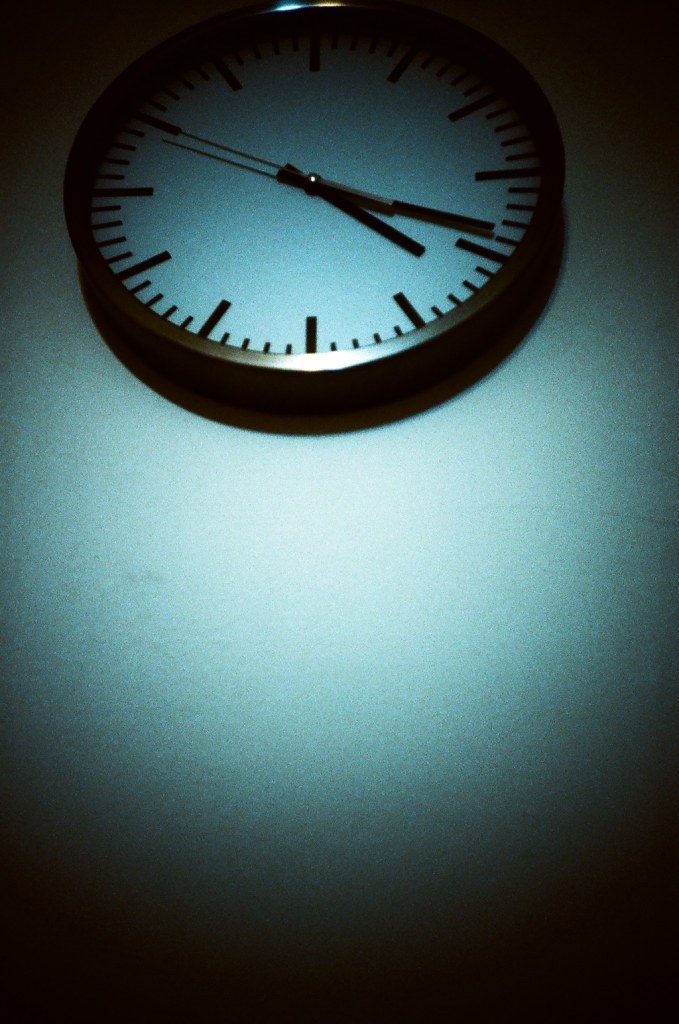In this striking image, we see a wall clock mounted on a muted white-gray wall. The photograph, taken from a slightly lower angle looking up, features a clock framed in chrome silver casing that projects slightly outward from the wall. The wall has an interesting lighting effect, casting an aqua green glow around the clock, which gives the clock face an aquamarine tint. 

The clock itself has a clean, minimalist design, with a white face devoid of numbers. Bold black lines indicate the hours, while shorter, thinner lines mark the minutes. The clock's hands are black, with a second hand in silver. Noteworthy is the translucent, almost floating appearance of the clock, making it seem as if the hands are mounted directly on the wall devoid of visible mechanics. Currently, the hands indicate a time around 3:14, although there are slight discrepancies in the timing observed. The distinctive corners of the image are shadowed in black, adding to the intriguing play of light and shadow.